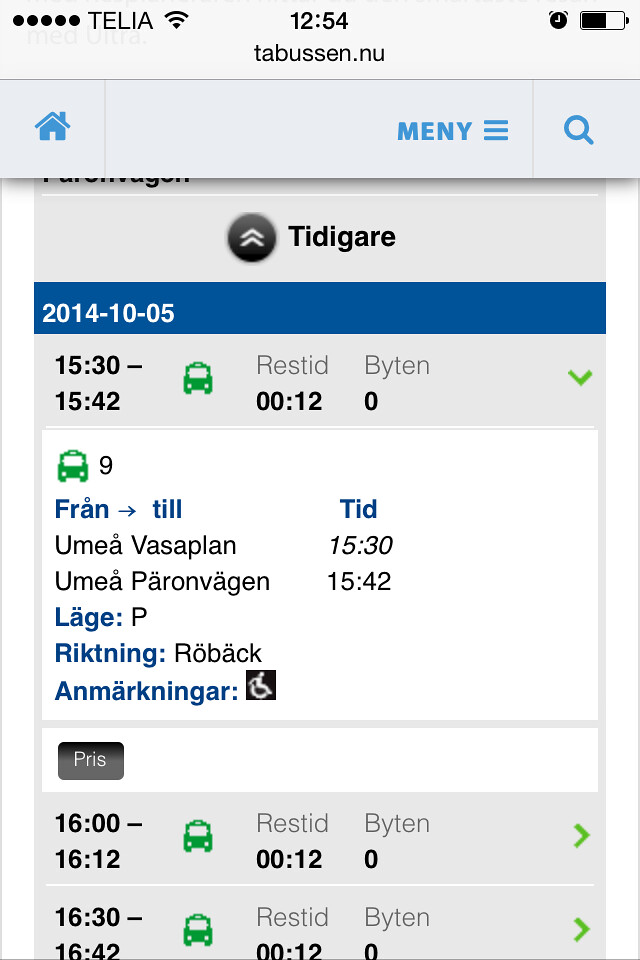This detailed color photograph captures a screenshot of a bus schedule displayed on a digital device, set against a light gray background. At the top, there is a small house icon representing the home button, beside the blue letters "MENY," indicating the menu. A black font displays "TIDYGARE," while a dark blue strip features the date "2014-10-05." Below, the schedule is detailed in a foreign language, possibly Eastern European or Latin American, showcasing various bus route options with corresponding times. The schedule prominently features several small green bus icons, likely indicating bus routes. A white center panel lists destinations next to the bus times. Additionally, the screen includes a small handicap symbol, enhancing accessibility. The captured details include dynamic blue bars highlighting key information and various small green bus icons denoting specific routes or bus services.